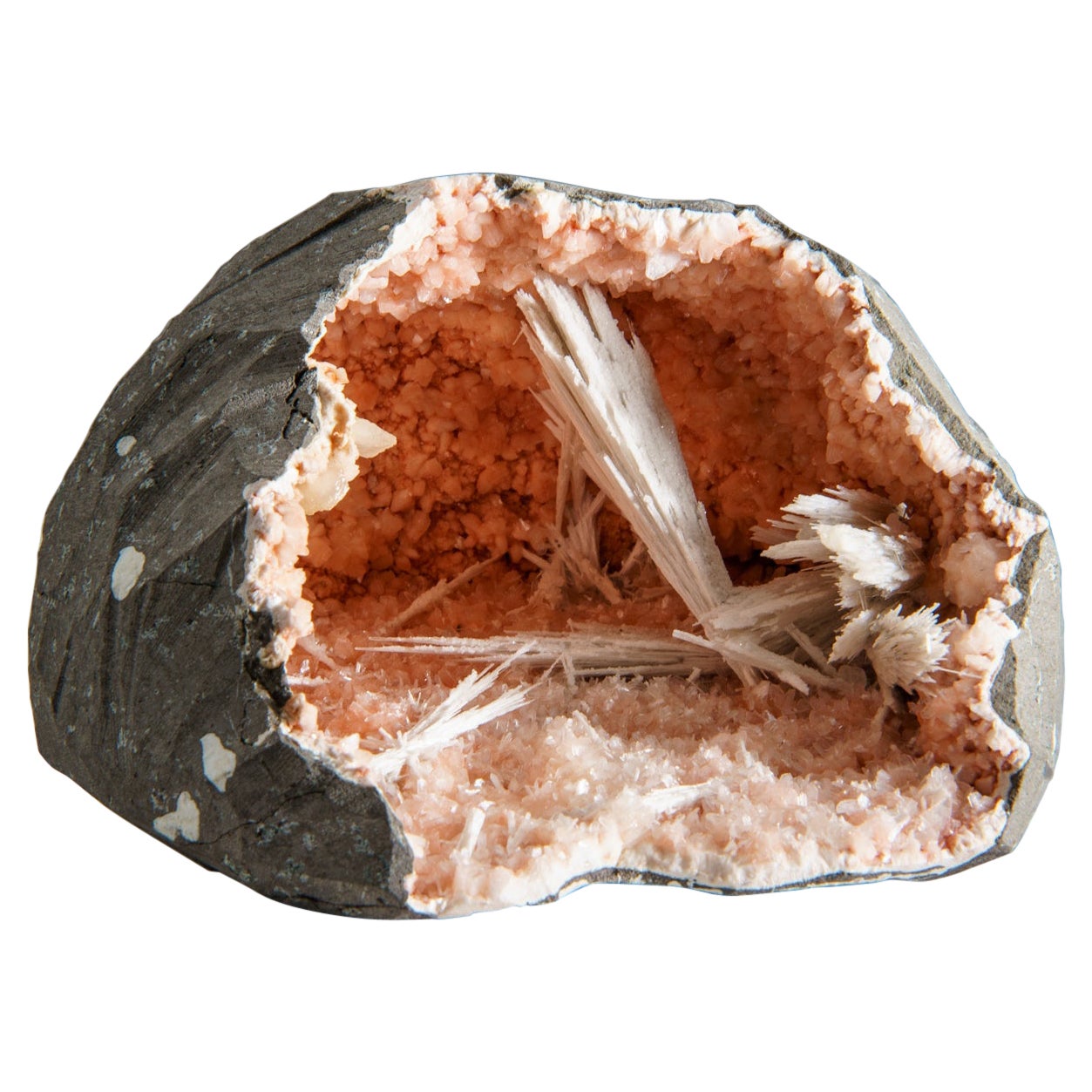This photograph captures the interior of a geode, displayed against a solid white background. The geode's exterior features a gray crust speckled with light blue and lighter gray spots. The front face is broken open, revealing a captivating interior of bright pink crystals. The majority of the pink crystals are small and bumpy, lining a large central void, while some exhibit long, spear-like formations. These slender, whitish crystals primarily jut out from the lower right side, extending from the bottom to the top of the geode in various angles. The overall impression is of a pink-hued crystalline landscape within the geode's rugged gray exterior.